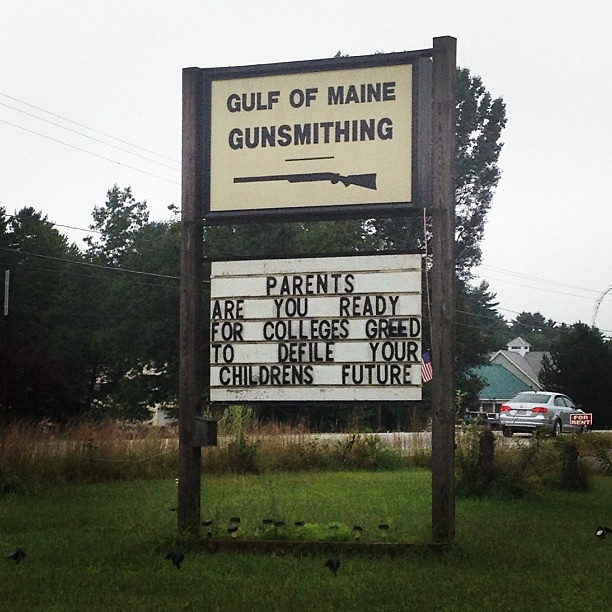In this photograph, taken on an overcast day, a prominent wooden sign stands in a lush, green lawn bordered by bushes and tall, dark green trees. The sign is composed of two sections: the top portion is a white rectangular board with black text reading "Gulf of Maine Gunsmithing" above a black illustration of a rifle. Below this, the sign holds a black and white marquee with a provocative message that states, "Parents, are you ready for college's greed to defile your children's future?" At the corner of the sign, a small American flag is attached. The background reveals a country road with a silver Volkswagen sedan passing by, and residential houses are visible in the distance. Additionally, lights or spotlights are mounted in the grass to likely illuminate the sign at night. A "for rent" sign can be seen beside the car, under a light gray sky.